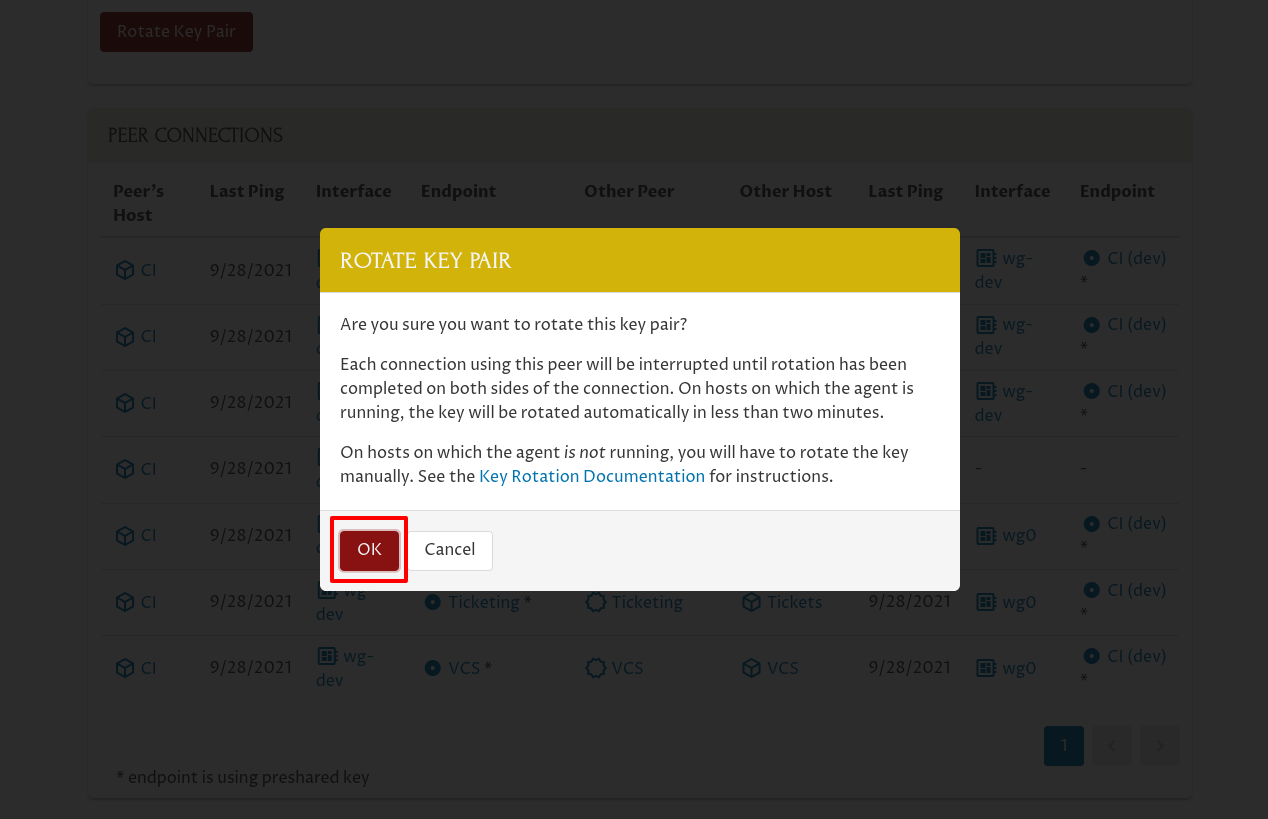The image is a rectangular screenshot with the long side stretching from left to right. The majority of the background displays a dark grayish-black color through which a faint background of a spreadsheet or table can be seen with a header running horizontally and columns extending vertically.

Dominating the image is a pop-up window that has an orangey-brown border along the top edge. The banner on this pop-up has the text "Rotate Key Pair" written in white. Below this banner, the main section of the pop-up has a white background with black text. The message displayed reads:

"Are you sure you want to rotate this key pair? Each connection using this peer will be interrupted until rotation has been completed on both sides of the connection. On the host where the agent is running, the key will be rotated automatically in less than two minutes. On the host where the agent is not running, you will have to rotate the key manually. See the key rotation documentation for instructions."

At the bottom of the pop-up window, there are two buttons. The first button is a red rectangle with white text that says "OK," which is further highlighted by another red box around it. The second button is a white rectangle with black text that says "Cancel."